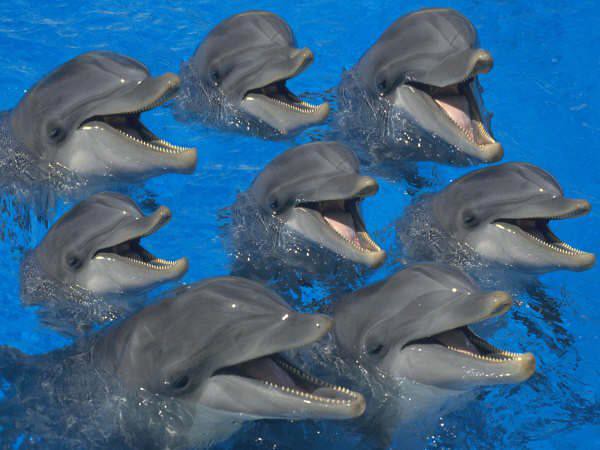In this vibrant color photograph, we see a close-up image of eight dolphins emerging from very clear, bright blue water, likely from a pool in an aquarium or zoo setting. The high clarity and vividness of the water hint that it may have been digitally enhanced or photographed on a very sunny day. Aligned in rows, the dolphins are predominantly facing in the same direction, offering mostly side profiles. Their medium to silver-gray heads are the most visible part, with the rest of their bodies disappearing beneath the water’s surface. Each dolphin has its mouth wide open, revealing small, sharp, razor-like teeth, and some display pale pink tongues. Interestingly, their eyes appear to be closed, adding to a cheerful and jolly demeanor.